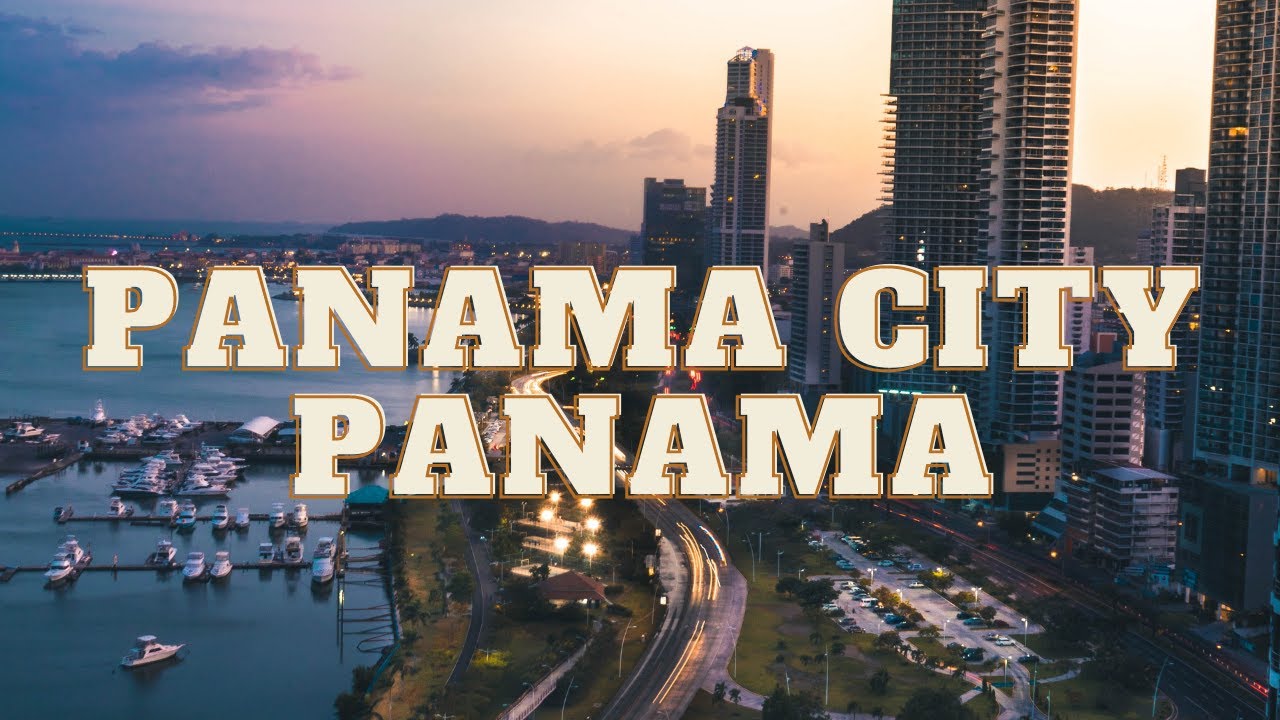This captivating image, a panoramic view of Panama City, presents a breathtaking high-altitude perspective capturing the essence of urban and natural beauty. To the left, a deep blue body of water provides a tranquil backdrop, where numerous boats are moored in the bottom left corner, adding a touch of liveliness to the serene expanse. The scene is framed by distant hills silhouetted against a striking dark grayish-orange sky, punctuated with scattered clouds.

Dominating the bottom middle of the image is a bustling road, illuminated by the dynamic white streaks of light from the headlights of moving vehicles, indicating the city's vibrant activity. On the right side, an impressive array of tall skyscrapers and various buildings stands majestically, symbolizing the city's modern architectural prowess.

The center of this visually stunning image features bold, large block letters declaring "Panama City," with "Panama" subtitled beneath. The text is strikingly white, accented with a light brown border, ensuring it stands out against the cityscape.

This wide-format image captures the harmonious blend of natural and urban elements, devoid of any visible people, animals, airplanes, or helicopters, focusing purely on the sprawling metropolis and its enchanting surroundings.